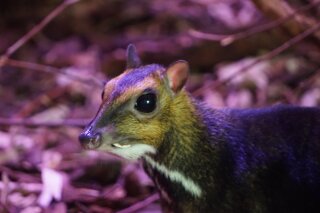The image depicts a small, nocturnal mammal resembling a cross between a large rodent and a member of the deer family. The creature stands out with its striking large black eyes and small, squat ears. Its pointed nose juts slightly forward, giving it a distinctive profile. The animal's coat is a dark brown with lighter fur around the face, a white stripe running from its neck, and white fur underneath its chin and on its chest. It possesses two fang-like teeth protruding from either side of its mouth and appears to be holding something that looks akin to a feather. The background is a forest floor scattered with twigs, leaves, and small limbs, partially blurred to emphasize the animal. The lighting suggests it is nighttime, possibly highlighting the animal's nocturnal nature, with some parts of its fur in shadow and hints of purplish light.